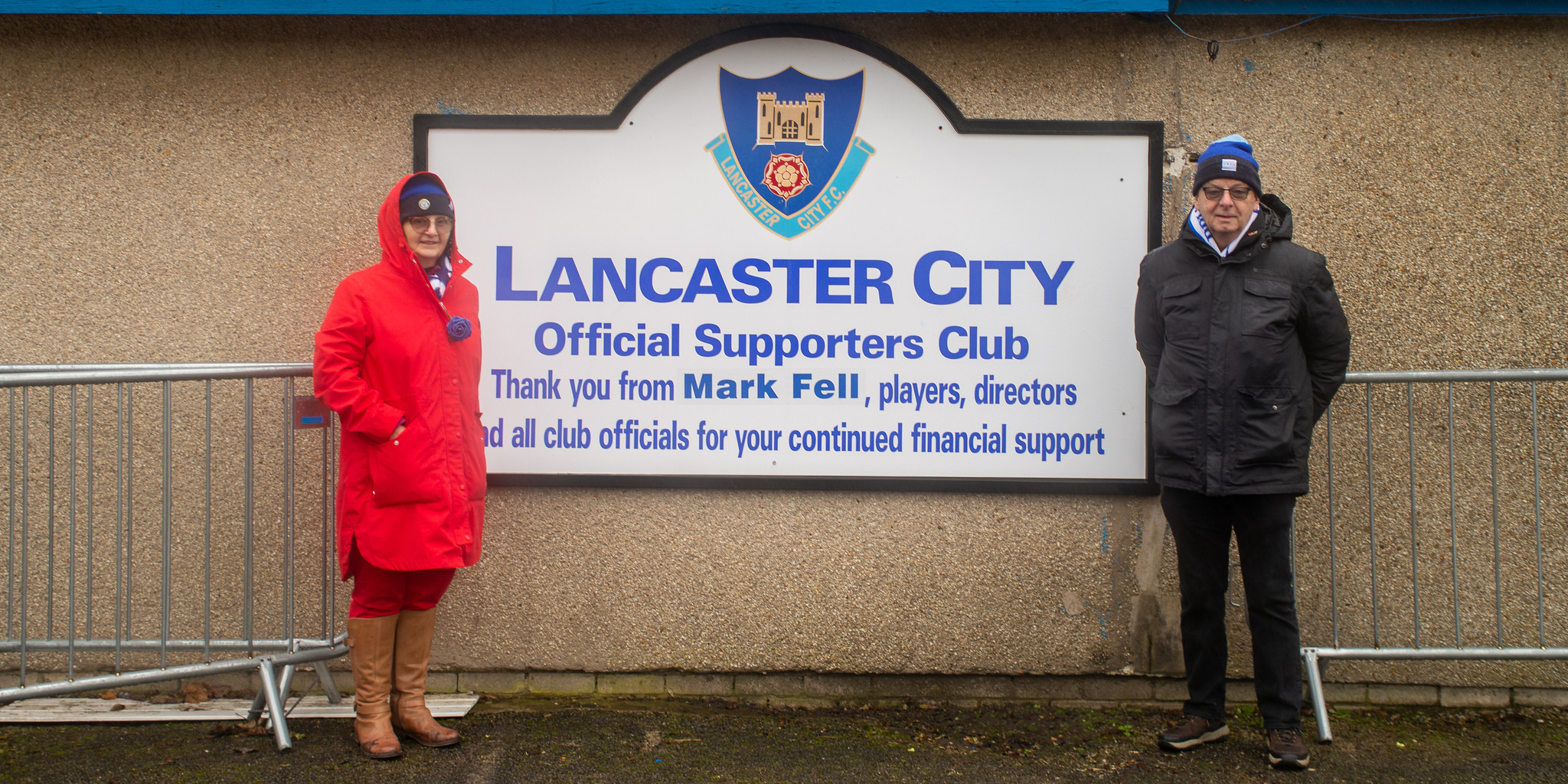In this detailed photograph, two individuals, a man and a woman, stand on either side of a prominently displayed sign mounted on a textured tan concrete wall. Two silver metal gates flank the image on the left and right, and the ground beneath them looks like dirt. The sign is rectangular with a slight oval bump at the top, and below this bump, it features a blue shield with the emblem of a castle and a fireball, signifying Lancaster City FC. Centered in the image, the sign reads, "Lancaster City Official Supporters Club. Thank you from Mark Fell, players, directors, and all club officials for your continued financial support."

The woman on the left wears a red jacket, a red coat, a blue beanie, glasses, and tan boots, while the man on the right is dressed in a blue jacket, dark black pants, and a blue and black beanie. He also sports glasses. The setting appears to be outdoors, likely mid-day, suggesting they are standing outside a club or official building. The colors in the image include light blue, tan, black, white, red, gray, and yellow, adding vibrancy to the scene.